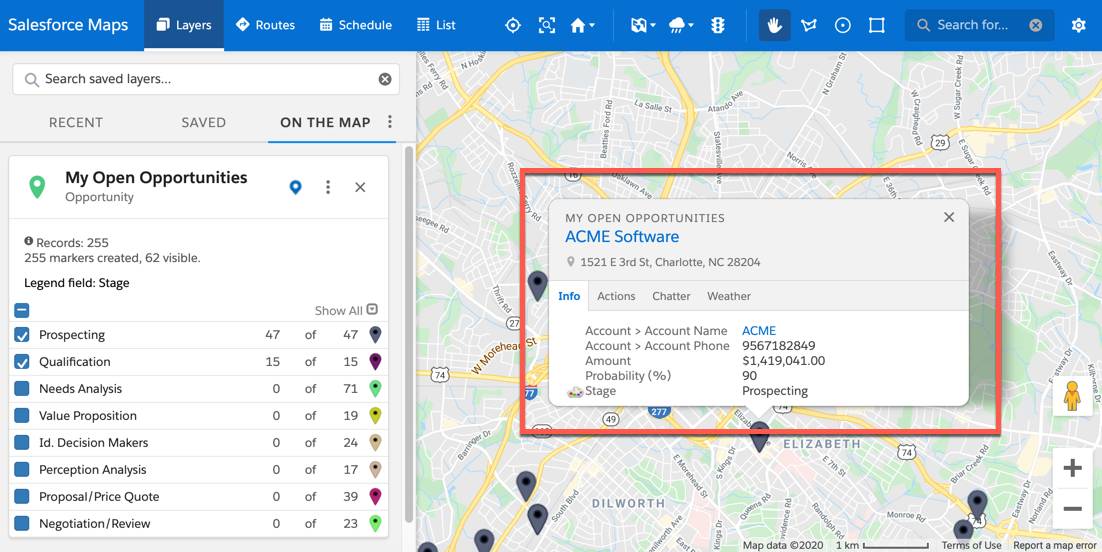This image features a screenshot of the Salesforce Maps website, clearly identified by the name "Salesforce Maps" displayed in the upper left-hand corner. The interface includes various tab options such as "Layers," "Routes," "Schedule," and "List," with the current selection being the "Layers" page.

Below the tabs is a search bar labeled "Search Saved Layers," accompanied by options categorized as "Recent," "Saved," and "On The Map," with "On The Map" currently selected. Under these options, there's a section titled "My Open Opportunities," detailing various records. Specifically, it shows "Record 255," with 255 markers created and 62 visible. A legend field named "Stage" is visible, offering stages like "Prospecting," "Qualification," "Needs Analysis," "Value Proposition," "ID Decision Makers," "Perception Analysis," "Proposal/Price Quote," and "Negotiation/Review."

On the right-hand side of the screen, there is a prominent red rectangle containing "My Open Opportunities - Acme Software," indicating specific opportunities related to the Acme Software firm.